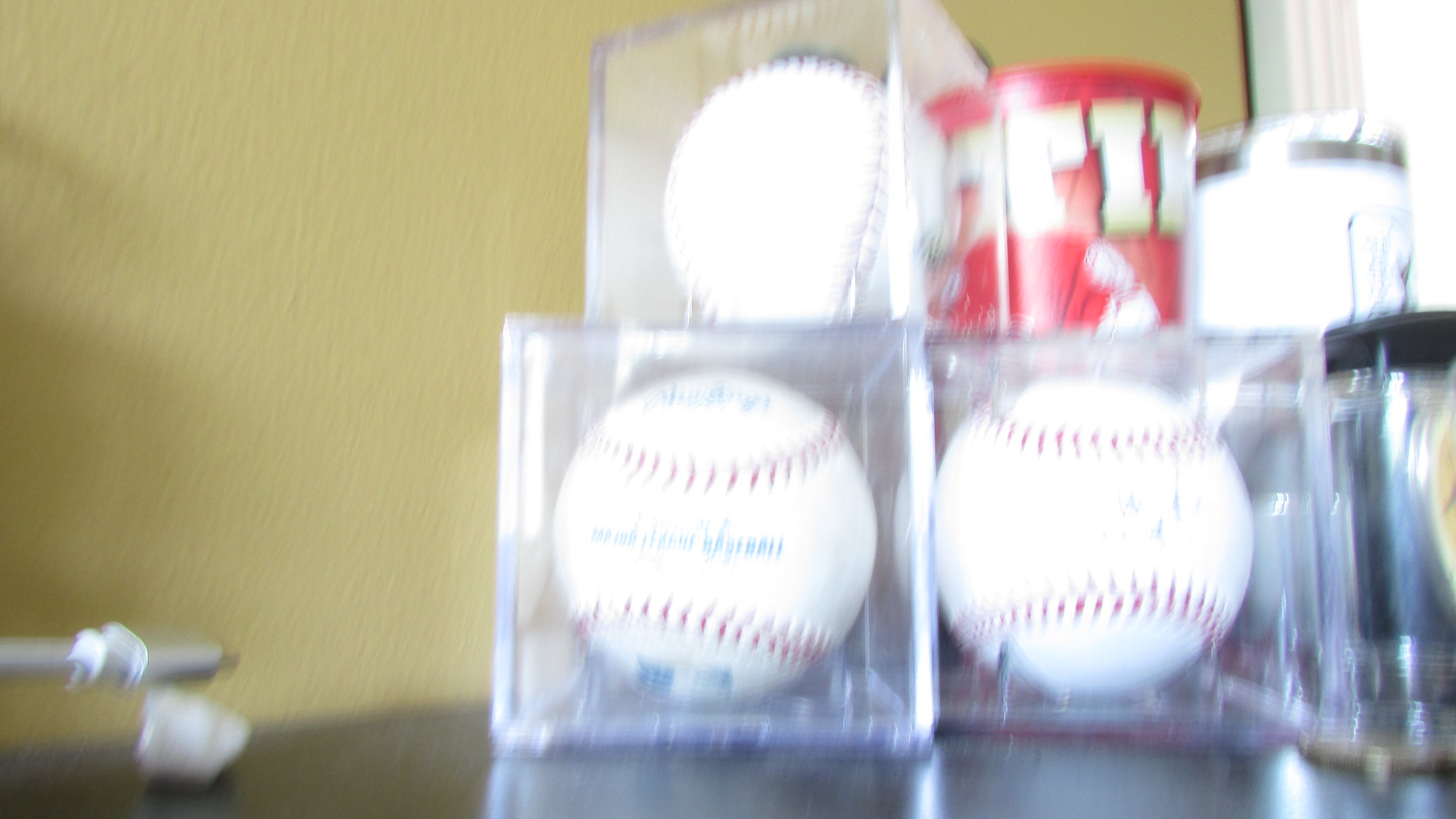In this out-of-focus, shaky photograph taken indoors, a brown countertop is visible against a green or tan-colored wall. Displayed prominently on the countertop are three baseballs, each encased in square, transparent glass or plastic containers, suggesting they are collector's items. These baseballs appear pristine, possibly bearing blue writing or autographs, though the text is indistinguishable due to the blur. The baseballs are organized into two rows: two containers at the bottom with one stacked on the left container. Next to the right container sits a red tin with unreadable text, likely for a product such as protein powder. Additionally, there is a white tin with a silver cap and a smaller glass bottle with a black screw cap positioned below the rightmost baseball. The overall setting suggests a display of valuable collectibles, carefully arranged despite the photograph's lack of clarity.